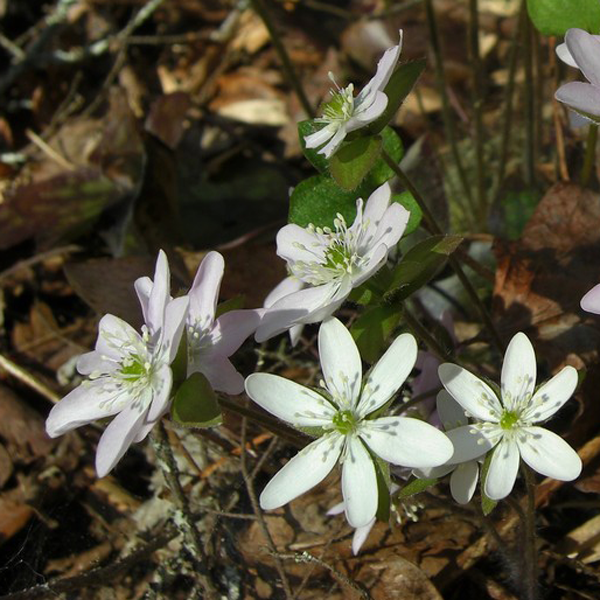This close-up image captures a cluster of delicate white flowers with oval petals, each flower comprising six petals arranged symmetrically around a vibrant green center. The green center is surrounded by lacy, elongated white stamens extending outward. The flowers, resembling horkelia or daisy-like blooms, are prominently positioned in the middle and lower portions of the square frame. They are anchored by fine, thin stems and a scattering of richly green, velvety leaves with faintly hairy edges. The background of the photo features blurred elements, including brown leaves, twigs, and forest litter, creating a stark contrast to the pristine white petals of the flowers. This scene suggests an early spring or late winter setting, where these flowers bloom amid dormant foliage and dead branches. In total, around half a dozen flowers are visible, indicating a small but vibrant patch of growth.